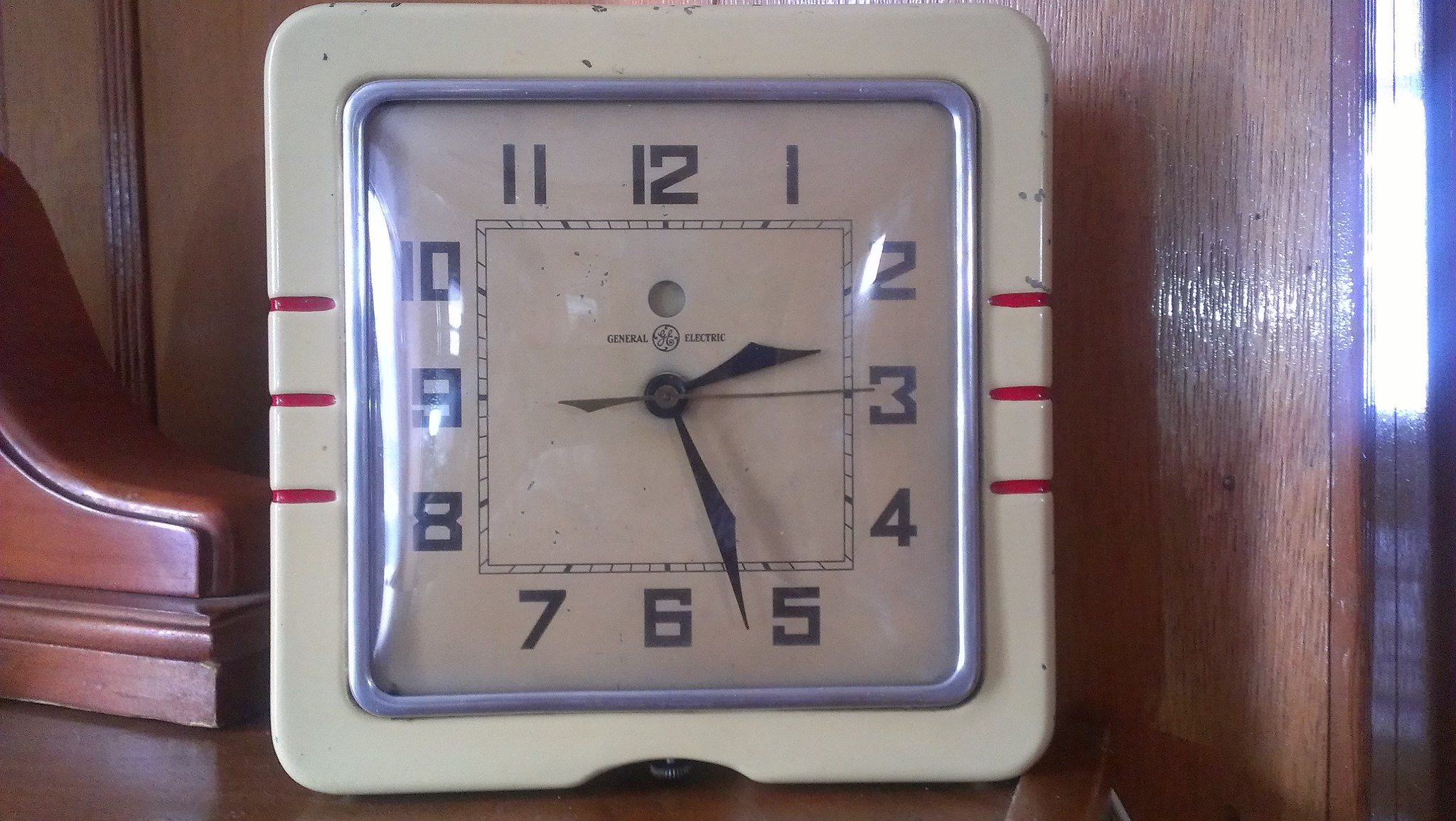This photograph features a square General Electric clock prominently placed at the center. The clock is framed by a white, enamel-like, or porcelain-like cover, adorned with three thin red stripes running vertically on each side. The main frame within the cover is a sleek silver-gray, encasing a glass-like front. Inside, the clock face is light-colored, possibly white, with bold black numbers marking 1 through 12 in a classic sequence. The hour hand is positioned just below the 2, the minute hand is just past the 5, and the second hand is also black. The inscription inside the clock reads "General Electric" with the iconic company logo centrally placed. The entire scene is set on a wooden table, with wood paneling visible in the background, adding a warm, rustic touch to the composition.